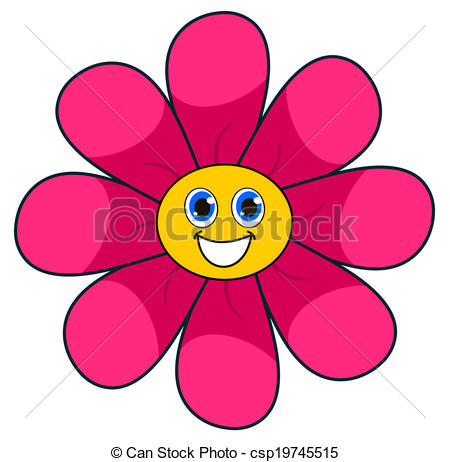The image is a colorful, retro-style cartoon of a flower featuring eight prominently outlined petals in varying shades of pink with darker tones toward the center. Nestled at the heart of the flower is a yellow, slightly oval-shaped center with a cheerful face, characterized by large blue googly eyes and a big white smile. The entire drawing is distinctly outlined in a thick black line, enhancing its vibrant, cartoony appearance. The image includes a gray watermark that reads "CanStock" alongside a camera icon with a gray X, along with the text “Canstockphoto-CSP19745515” and the copyright symbol in small black letters at the bottom. The background is white, highlighting the playful and cute aesthetics of the flower.